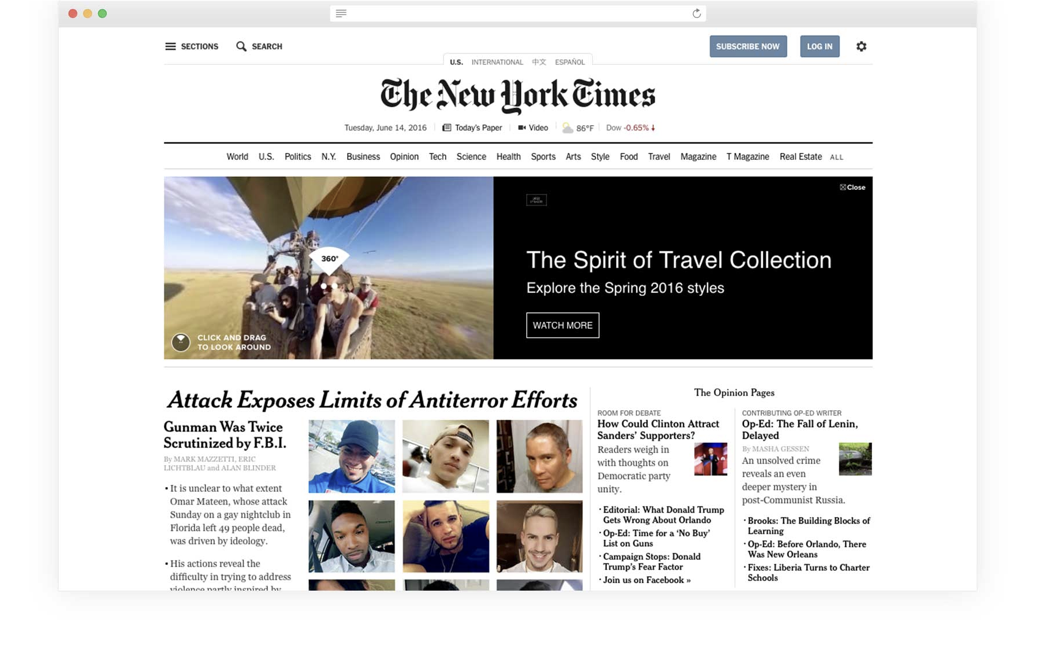This image depicts the homepage of The New York Times as of Tuesday, June 14, 2016. Central to the design is the iconic New York Times title, rendered in a traditional old English script, giving it an artistic and timeless feel. The background is predominantly white, creating a clean and readable interface, with most of the text in black. Below the date, a black menu strip features various categories including World, U.S., Politics, New York, Business, Opinion, Tech, Science, Health, Sports, Arts, Style, Food, Travel, Magazine, T Magazine, Real Estate, and All.

Prominently displayed are previews of highlighted articles. One featured article, "The Spirit of Travel Collection," is set against a black rectangular background with white text. Next to it, a vibrant image shows several individuals in a hot air balloon basket, floating over a desert landscape under a bright blue sky dotted with clouds. 

Below, another article titled "Attack Exposes Limits of Anti-Terror Efforts" is accompanied by rectangular photographs of various people, possibly suspects or victims, providing a visual narrative to the headline. The right side of the homepage features additional articles from the Opinions section, ensuring a well-rounded representation of the day's news and views.